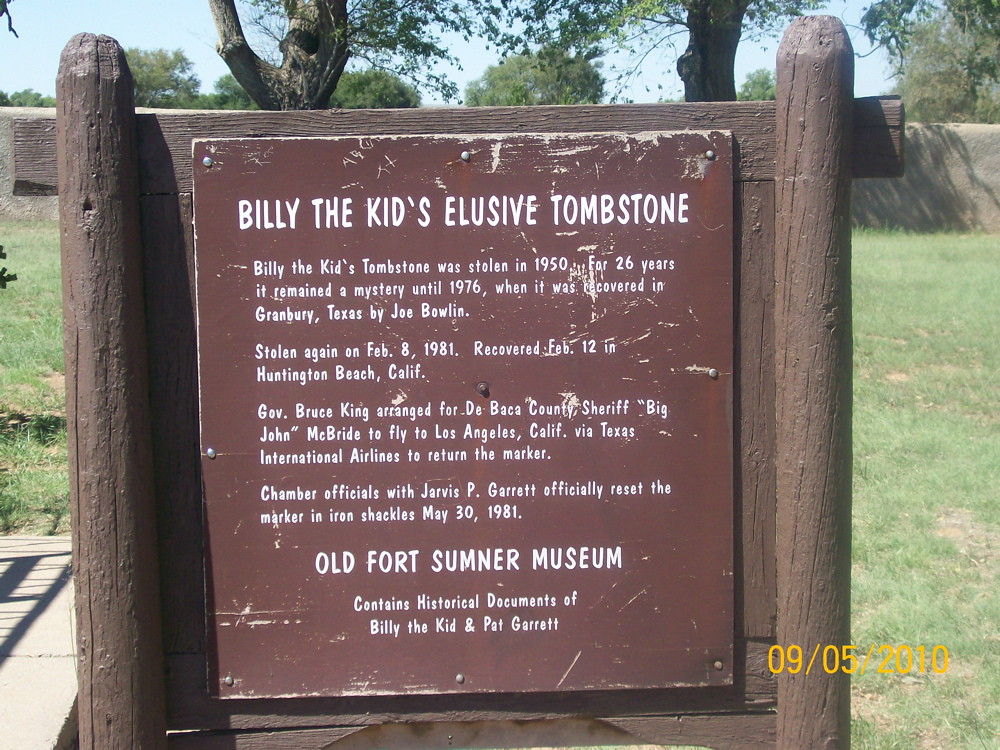This photograph, taken outdoors on September 5, 2010, captures a historical marker detailing the story of Billy the Kid's elusive tombstone. The marker, mounted on brown-painted wooden posts with crossbeams, stands amidst a grassy field with trees in the background under a blue sky. The black painted sign is engraved with white text, bearing the title "Billy the Kid's Elusive Tombstone." The text narrates the turbulent history of Billy the Kid's tombstone, which was stolen in 1950 and remained missing for 26 years until it was recovered in Granbury, Texas by Joe Bolin in 1976. It was stolen again on February 8, 1981, but was found just four days later in Huntington Beach, California. Governor Bruce King facilitated its return to DeBaca County, New Mexico, with the help of Sheriff Big John McBride, who flew to Los Angeles via Texas International Airlines. Chamber officials, alongside Jarvis P. Garrett, reset the marker in iron shackles on May 30, 1981. The marker also mentions that the Old Fort Sumner Museum houses historical documents related to Billy the Kid and Pat Garrett. Despite some visible scratches on the plaque, this outdoor display remains a significant testament to a piece of wild west history.